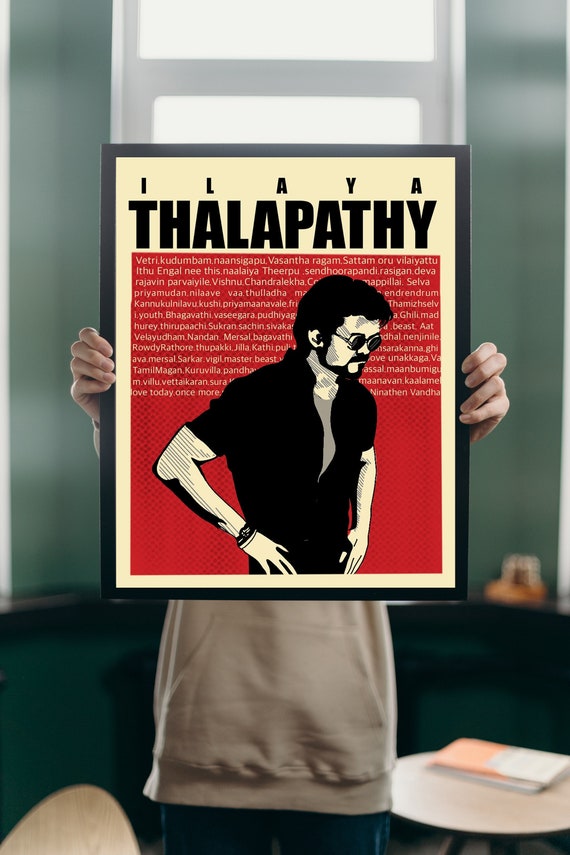In this image, a person is holding up a picture with both hands, framing it firmly between their fingers. The individual remains anonymous as their face is not visible, but they are dressed in a tan hoodie sweatshirt. Contextually, the person appears to be standing in a setting that resembles either a classroom or a library, suggested by the visible window and the general ambiance of the room.

The picture they are presenting features a man with a confident stance—his hands resting on his hips, wearing sunglasses, and sporting a beard. Above this striking figure, the name "ILAYA" is inscribed in smaller, evenly spaced black capital letters. Directly below, in larger block capital letters, the last name "THALAPATHY" spans the width of the picture. The entire text is set against a bold red background, making the letters and the image of the man stand out prominently.